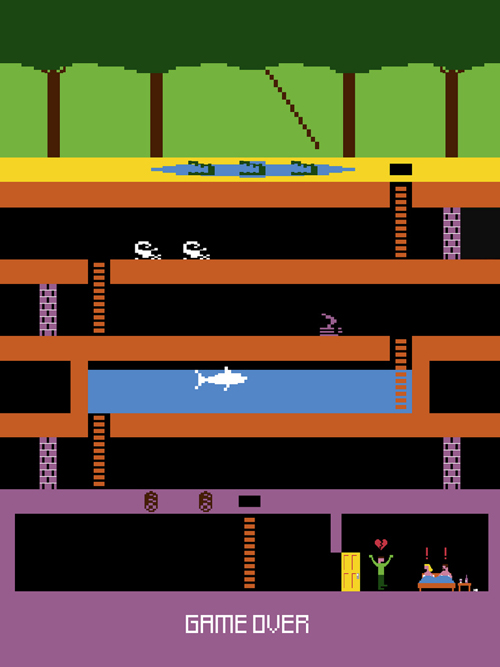The image is a detailed screenshot from a retro video game, featuring simple colors and shapes characteristic of early arcade games. At the top, there is a vibrant forest scene with a small pool containing crocodiles. Below the forest, the game transitions into an underground area with multiple horizontally-aligned levels connected by ladders. The center of this underground area includes a pool inhabited by sharks. The lowest part of the image showcases a distinct purple subterranean section with a yellow door through which a character has just entered. This character, with something red above their head, encounters two people in bed with blue sheets, and an end table adjacent to them holding two items. The bottom of the screen prominently displays the text "Game Over," reminiscent of old coin-operated video games like Pac-Man, and signifies the end of the game.